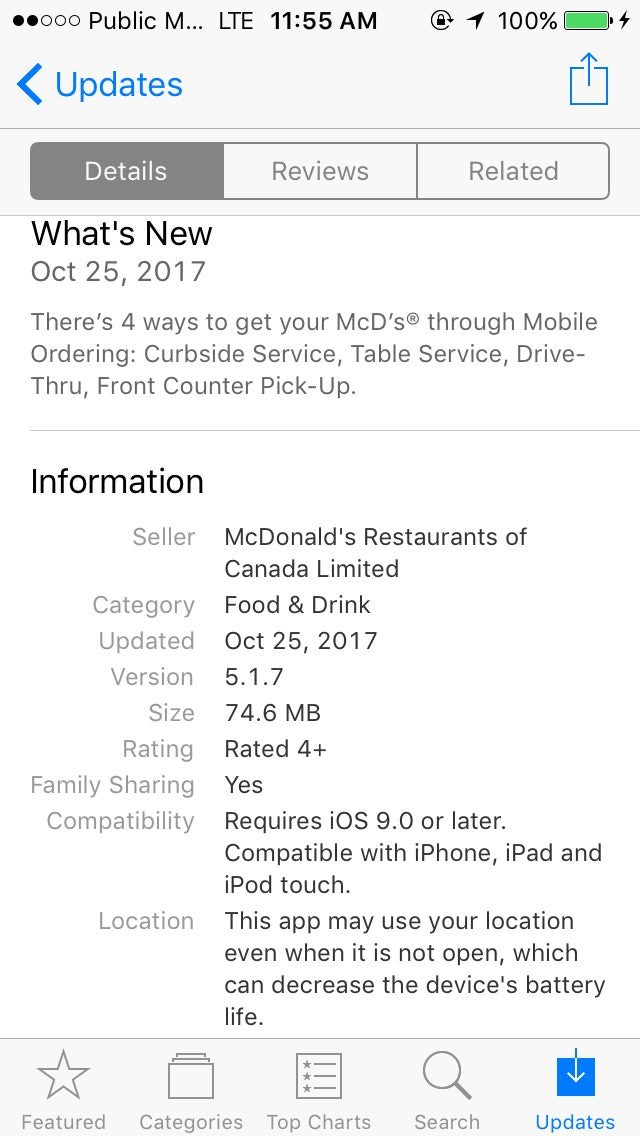A screenshot from a cell phone taken at 11:55 a.m. showcases the detailed information page for the McDonald's app on the App Store. At the top of the screen, there's a lock icon with a circular arrow around it and a location tag, indicating the user's phone has a 100% battery. The screen shows the app listing under "Public M..." followed by two solid circles and three outlined circles at the top.

Highlighted is the "Details" tab in gray with white font. Below, it specifies "What's New," dated October 25, 2017. The description highlights four ways to get your McDonald's: through mobile ordering, curbside service, table service, drive-thru, and front counter pickup. 

Under the "Information" section, it states McDonald's Restaurants of Canada Limited, categorized under Food & Drink. It details the last update on October 25, 2017, with version 5.1.7, a size of 74.6 MB, a rating of 4+, and indicates that family sharing is enabled. Compatibility requires iOS 9.0 or later, making it compatible with iPhone, iPad, and iPod touch. A note mentions that the app may use your location even when not open, potentially decreasing battery life.

At the bottom of the screen, there are options to navigate between "Updates," "Search," "Top Charts," "Categories," and "Featured." This screenshot captures a comprehensive view of the McDonald's app's presentation on the App Store.